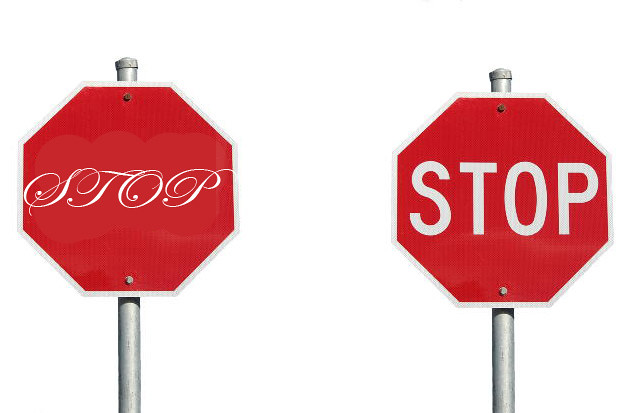The image showcases two stop signs against a plain white background, each mounted on a silver post that ends with a small rounded cap at the top. Both signs are red octagons with a white border, attached to the post with two nails each—black at the top and silver at the bottom. The sign on the right is designed in the classic style, featuring bold, white capital letters that spell out "STOP" in a plain font. In contrast, the sign on the left presents "STOP" in a fancy, cursive script where the letters are slightly italicized and stylistically connected with multiple swirls, giving it a decorative appearance.